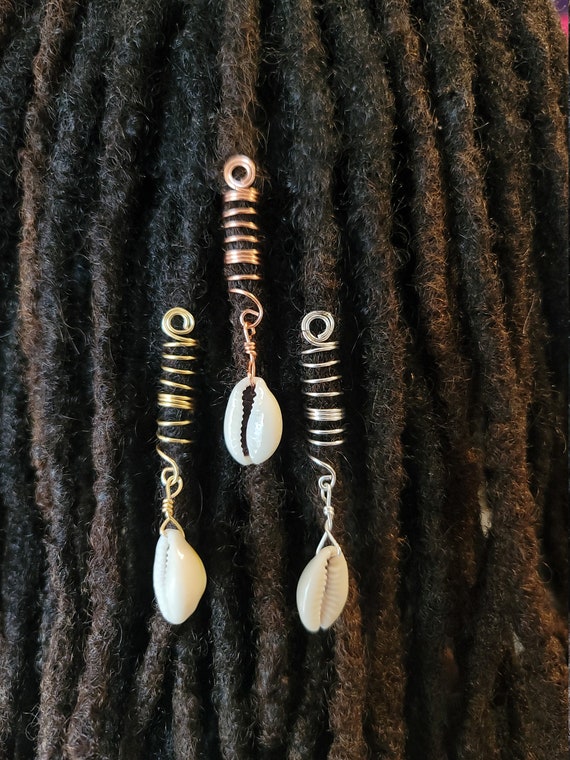The close-up photograph captures the intricate details of the back of someone's head adorned with tightly woven, long, thin dreadlocks of dark black and dark brown hair, with occasional streaks of lighter brown. Each dreadlock descends vertically, densely packed and filling the entire frame. Three notable pieces of jewelry are woven into the dreads at varying levels. Made primarily of coiled brass wire, the jewelry pieces each feature a small spiral at the top for decorative effect, with the wire wrapping neatly around the dreadlocks. Suspended from each coiled piece, there is a white seashell attached via a small hook and chain mechanism. These seashells hang at different heights across the central dreads. The background, discernible only in the upper right corner, suggests a hint of red, possibly indicative of a red wall. The overall composition highlights the artistic and cultural significance of the hair accessories against the rich texture of the dreadlocks.